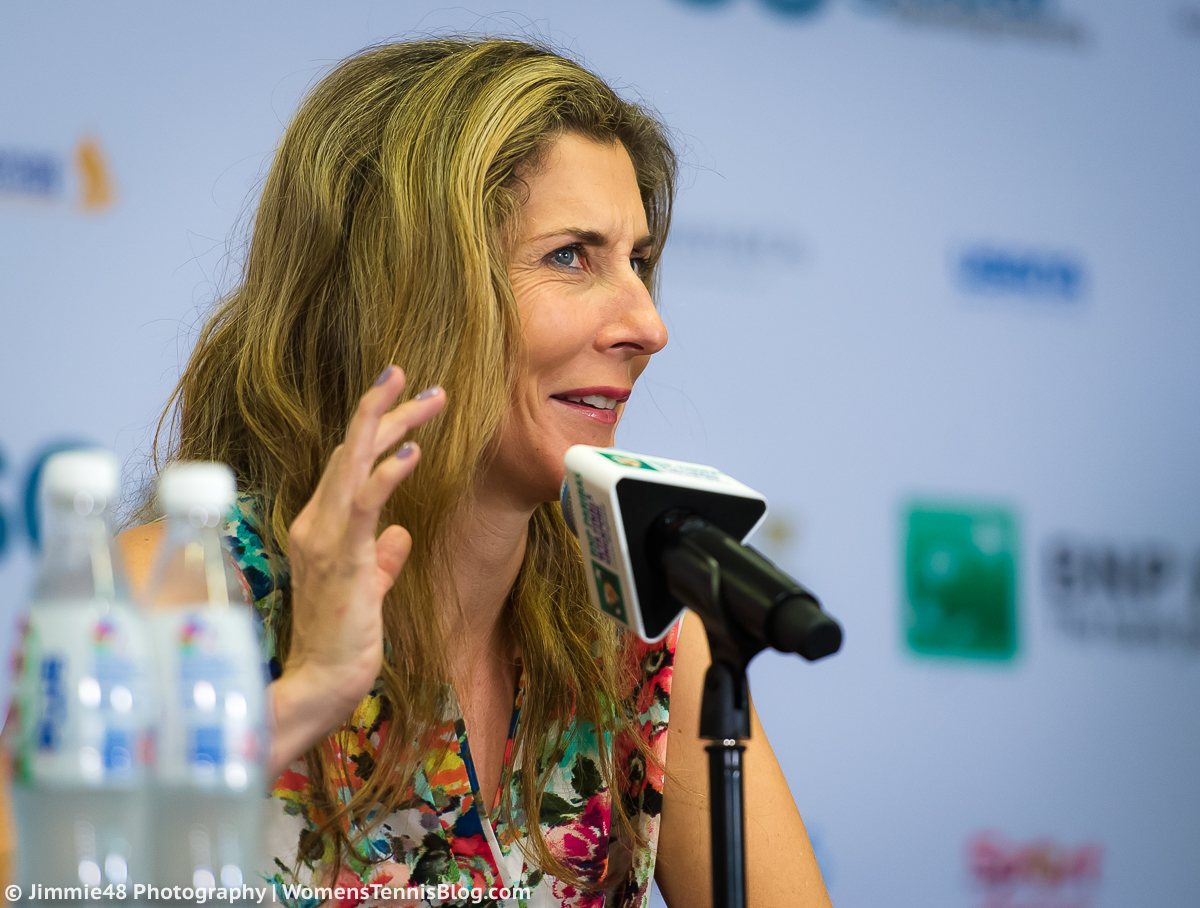The photograph captures a woman at a press meet, facing slightly right but looking upward towards the center. She is dressed in a vibrant, multicolored patterned dress featuring hues of yellow, orange, blue, pink, and green. Her dark hair is highlighted with yellow streaks, and she sports purple nail polish. In front of her is a black microphone with a triangular top displaying a logo. Her blue eyes and slightly prominent nose are noticeable, along with wrinkles around her eyes. The scene's bottom left shows two slightly out-of-focus water bottles. The background features a blurry white banner filled with indistinct logos in various colors, including green, red, blue, and orange. Additionally, there is a watermark on the bottom left corner reading "Jimmy 48 Photography" and "womens-tennis-blog.com" in white text.